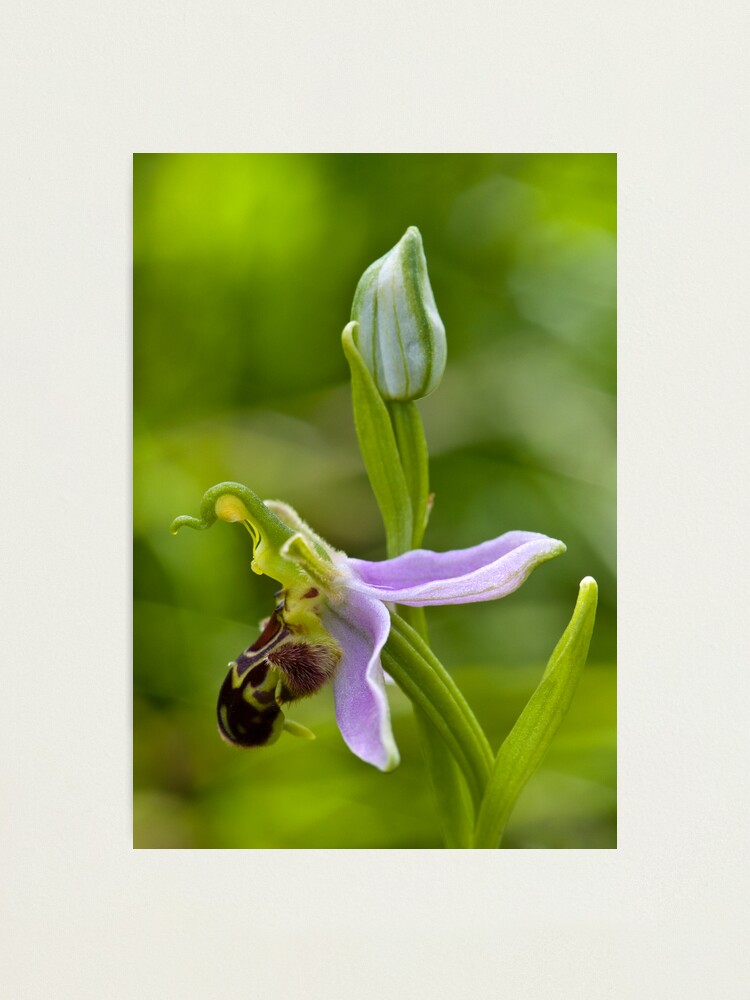The close-up image showcases a striking flowering plant, likely an orchid, against a blurred green and yellow backdrop evocative of a natural environment, possibly a forest or jungle. The main subject consists of a prominently bloomed flower displaying a captivating mix of lavender and dark purple petals, accented with variegated green and subtle yellow highlights. Adjacent to this bloom, another flower bud on a thick green stem waits to unfurl, its outer petals a pristine white veined with green. This bud, exhibiting a subtle grayish hue, adds a sense of anticipation to the scene, suggesting it might transform in color as it fully opens. The beautifully intricate details and contrasting colors of the flowers offer a vivid glimpse into the plant's unique blooming stages.